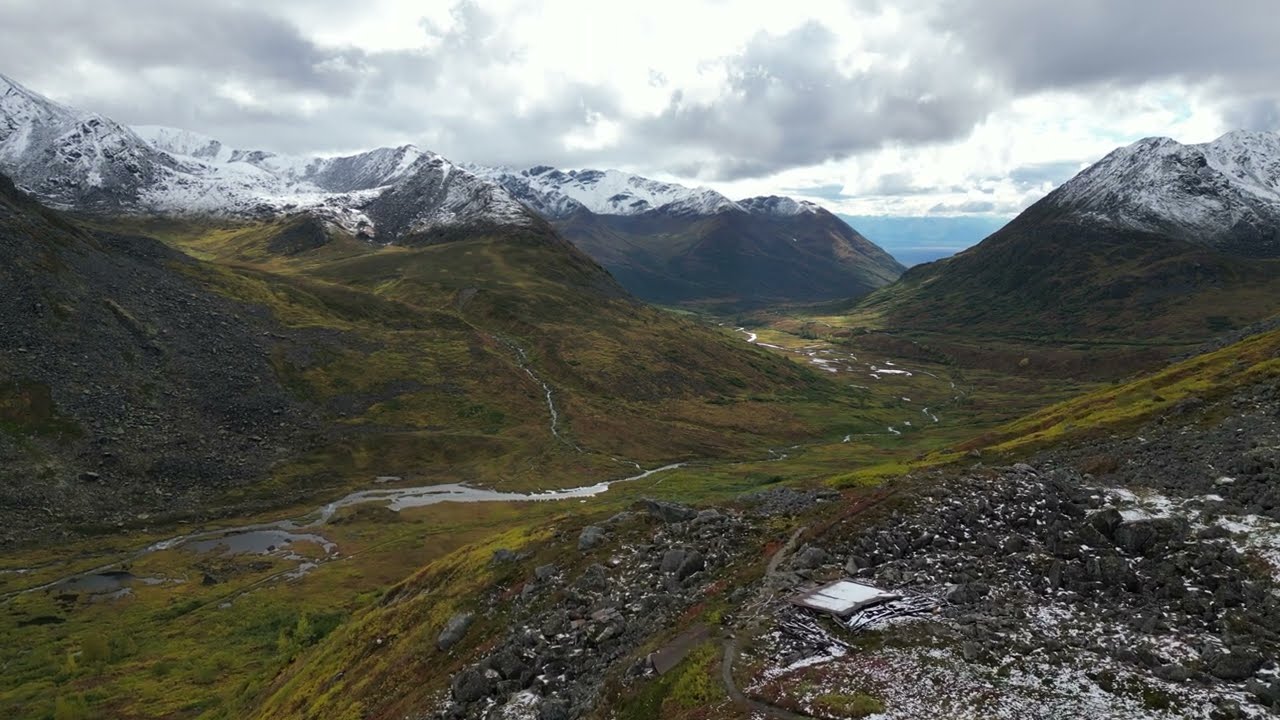This high-altitude landscape photograph captures a sweeping view of a mountainous region, where the white-capped peaks dominate the background, extending across the horizon. Majestic clouds, ranging from white to dark gray, envelop the sky, casting deep shadows over the scene and partially obscuring the sun, which peeks out for a moment through a break in the clouds. The valley below, in stark contrast, is free of snow and showcases a varied palette of light green and brown hues, reminiscent of moss and grass-covered terrain dotted with stones. A small river meanders through the valley, collecting into a pond on the left and bordered by snow in places where it seems to be melting. Scattered about the valley are a few modest dwellings. The foreground of the image is rocky with intermittent snow patches, further emphasizing the rugged yet serene beauty of the natural landscape.